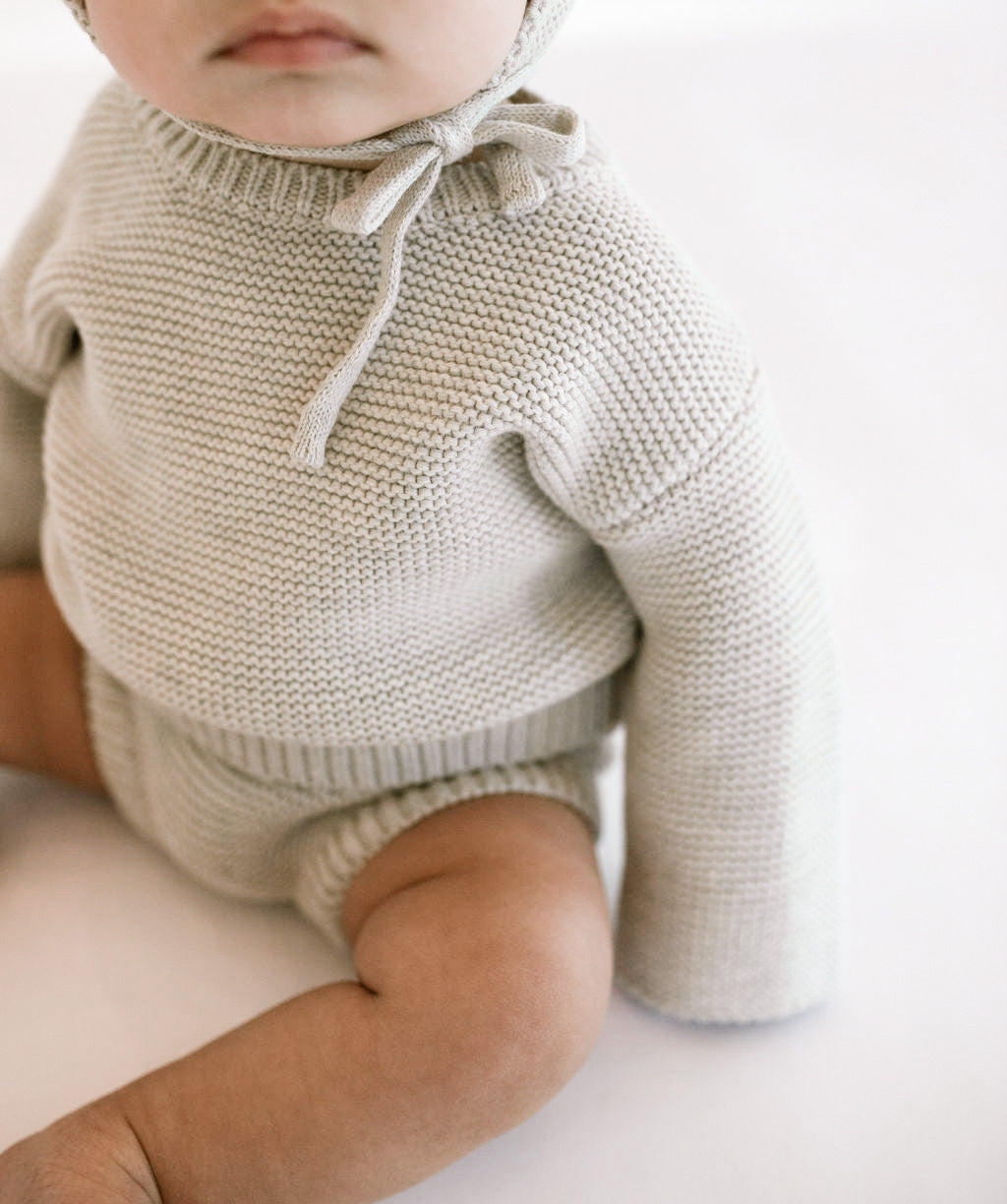The image features a chubby, pale-skinned baby sitting upright against a creamy white background. The baby appears to be around 2 to 12 months old, with its face partially visible and cut off just above the lips. The lips are pursed and downturned, giving the baby a contemplative expression. The baby is dressed in a matching knitted ensemble consisting of a light gray or cream-colored crochet-patterned sweater with long sleeves, and bloomers or shorts of the same material that end just above the knees. The baby is also wearing a bonnet or hat made from the identical crochet material, secured under its chin with long tied strings. One of the baby's legs is bent outward with visible rolls around the knee, while the foot is hidden in the left corner of the image. The overall setting and the baby's attire give a cozy, vintage feel to the photograph.